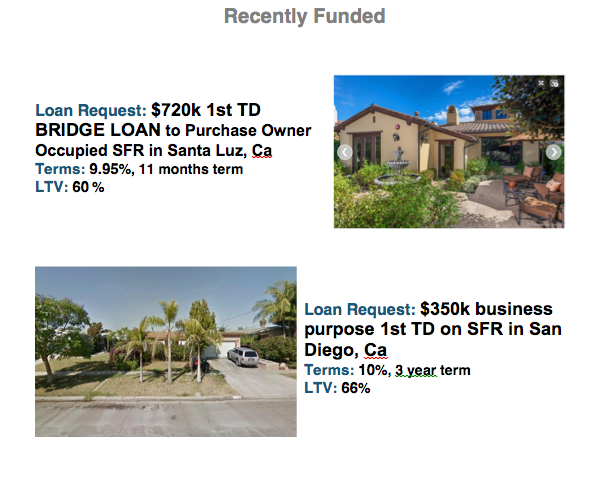Recently Funded Loan Approvals: Detailed Overview

1. **First Loan Request: Owner-Occupied SFR in Santa Luz, California**
   - **Loan Amount:** $720,000 (First TD Bridge Loan)
   - **Terms:** 9.95% interest rate, 11-month term
   - **Loan-to-Value (LTV) Ratio:** 60%
   - **Property Description:** The property is a grand, South American-style single-family residence (SFR) located in the upscale neighborhood of Santa Luz, California. The house features a large, elegant structure painted in a rich, yellowish hue, and includes multiple seating areas, lush grass, various plants, and an ornate fountain, highlighting its luxurious status.

![SFR in Santa Luz](link_to_image)

2. **Second Loan Request: Business Purpose SFR in San Diego, California**
   - **Loan Amount:** $350,000 (First TD Loan)
   - **Terms:** 10% interest rate, 3-year term
   - **Loan-to-Value (LTV) Ratio:** 66%
   - **Property Description:** Situated in San Diego, California, this property is more modest in comparison to the first. It is surrounded by palm trees, contributing to a tropical ambiance. While smaller and located in a less upscale area, the property enjoys a lush, tree-dense environment. The nearby road appears unpaved, adding a rustic feel to the otherwise verdant locale.

![SFR in San Diego](link_to_image)

Both properties reflect diverse yet noteworthy investments, each tailored to different market needs and loan parameters.